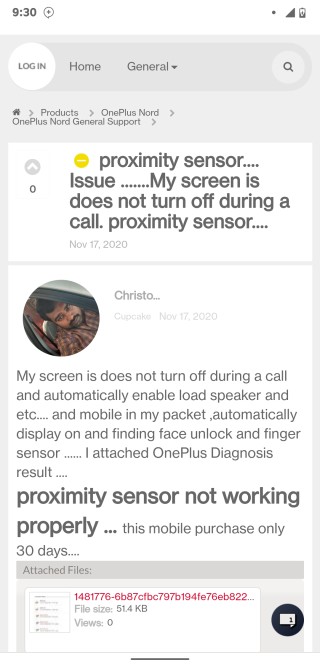Screenshot of a mobile phone screen displaying a complaint on a technical support forum. At the top, there is a white, circular "Login" button, followed by the headings "Home" and "General". Underneath, there are several navigation options including "Product", "Home", and "Products". The user navigates to "OnePlus Nord General Support".

A detailed post titled "Proximity Sensor Issue" is shown, dated November 17, 2020. The post, identified by a partial profile picture of a man named Christopher, reads: "My screen does not turn off during a call and automatically enables the loudspeaker. When my mobile is in my pocket, the display turns on automatically, triggering the face unlock and finger sensor. I have attached the OnePlus diagnosis results which indicate that the proximity sensor is not working properly. This mobile was purchased only 30 days ago."

At the bottom, there is an attached file with red text displaying diagnostic numbers. The attached file's size is 51.4 kilobytes and has zero views. A blue circle at the bottom right corner contains a speech bubble icon, with the number 1 inside it, indicating there is one comment on the post.